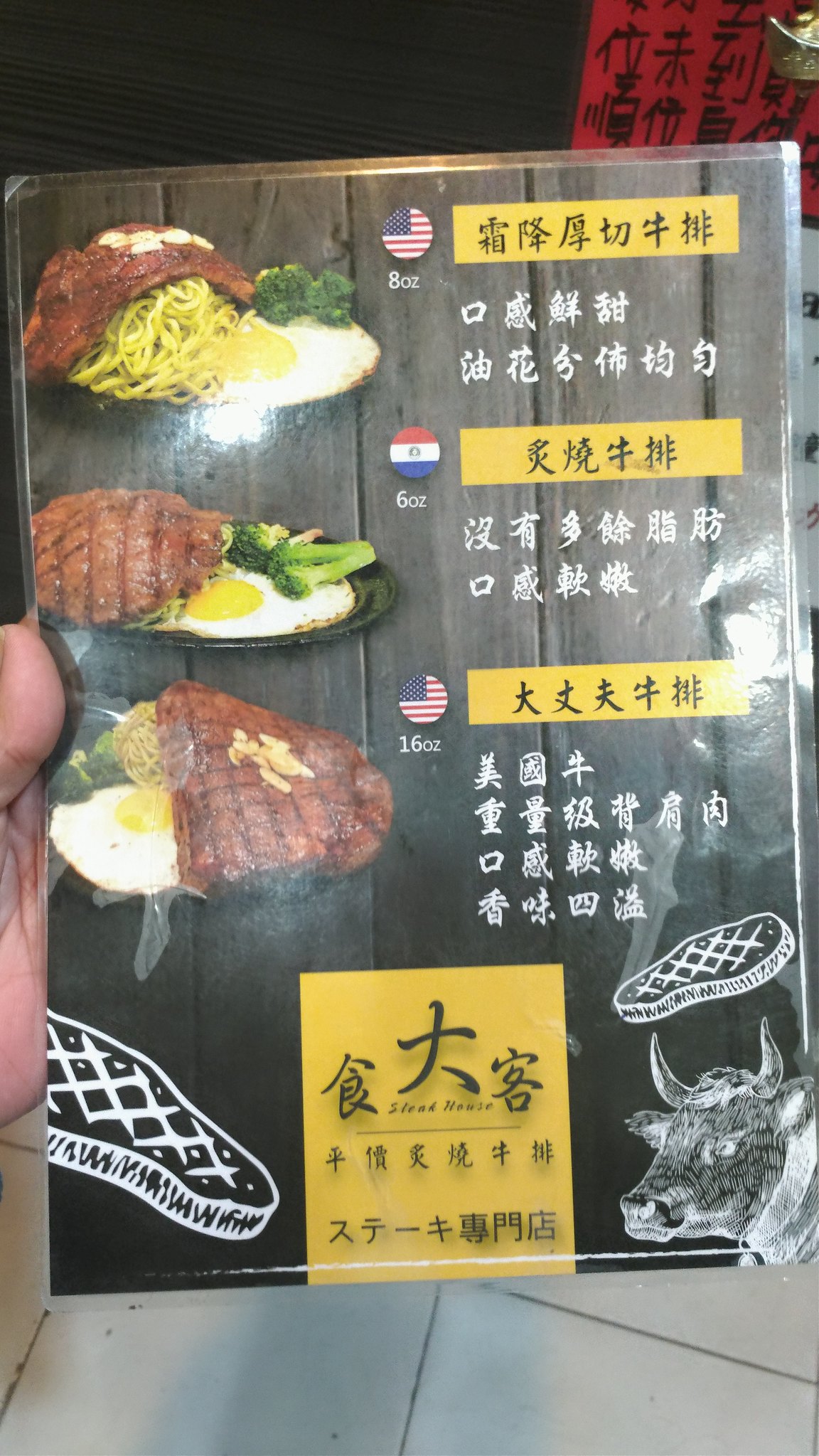The image appears to be an excerpt from a menu or a laminated card featuring a selection of steak dishes. At the very top of the card, the American flag is displayed next to some black text written in what seems to be Japanese, on a yellow background. Below this is another flag, accompanied by similar text, followed by the American flag with the same text once again.

To the left-hand side of the card, there are three different steak dishes depicted. The dish at the top includes a portion of steak served with noodles, steamed broccoli, and a fried egg. The dish in the middle appears to include only the steak and broccoli, omitting the noodles and egg found in the top dish. The dish at the bottom resembles the top one, featuring steak, noodles, broccoli, and a fried egg.